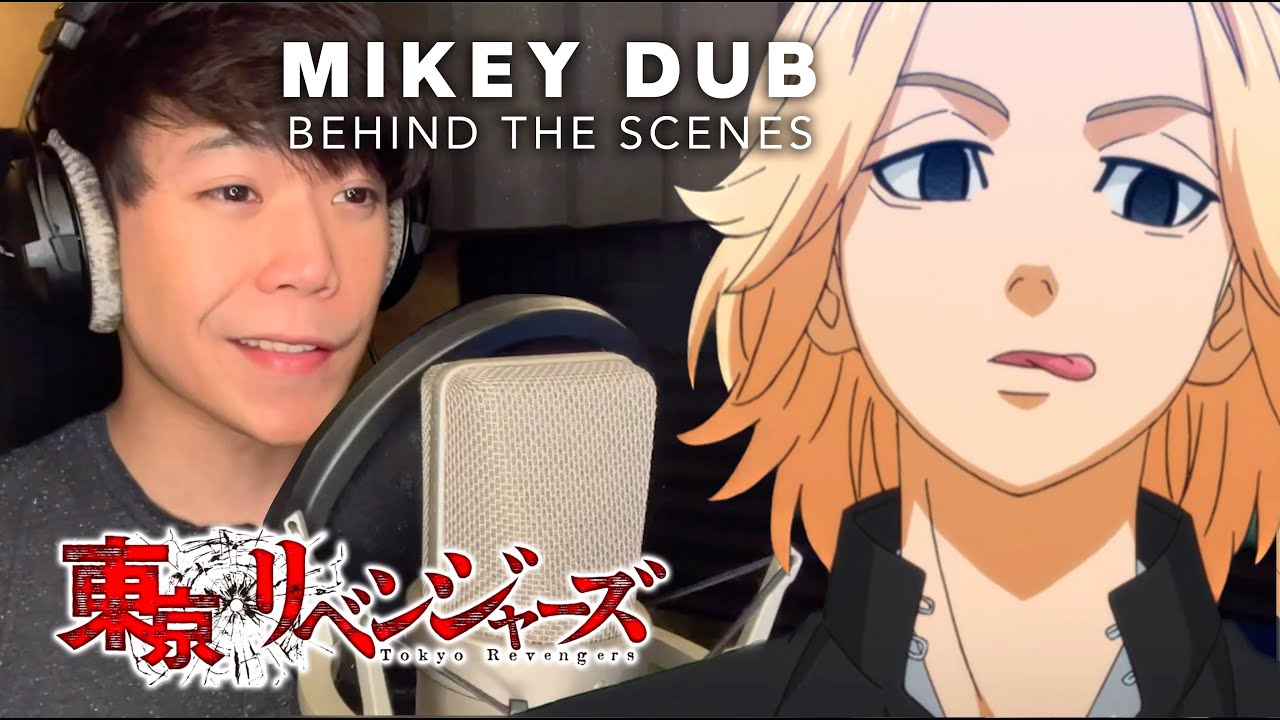In this detailed behind-the-scenes photo, we see Mikey Dub, an Asian man with brown hair, immersed in his voice recording session for the anime "Tokyo Revengers." Wearing over-the-ear headphones, Mikey speaks into a white microphone guarded by a pop filter. Positioned on the left side of the image, the text "Mikey Dub behind the scenes" appears, accompanied by Japanese characters that spell out "Tokyo Revengers." On the right side of the photo, there's an anime character with pale skin, blonde hair, and large blue eyes, styled in the traditional Japanese animation technique. The character's appearance, with a black jacket and blue shirt, suggests a certain intensity, further emphasized by their slightly protruding tongue. The color palette of the photo vividly includes red, silver, black, blue, white, yellow, and pink, lending an immersive and vibrant look to the scene. This snapshot captures the essence of Mikey actively bringing an animated character to life through his dedicated voice acting.